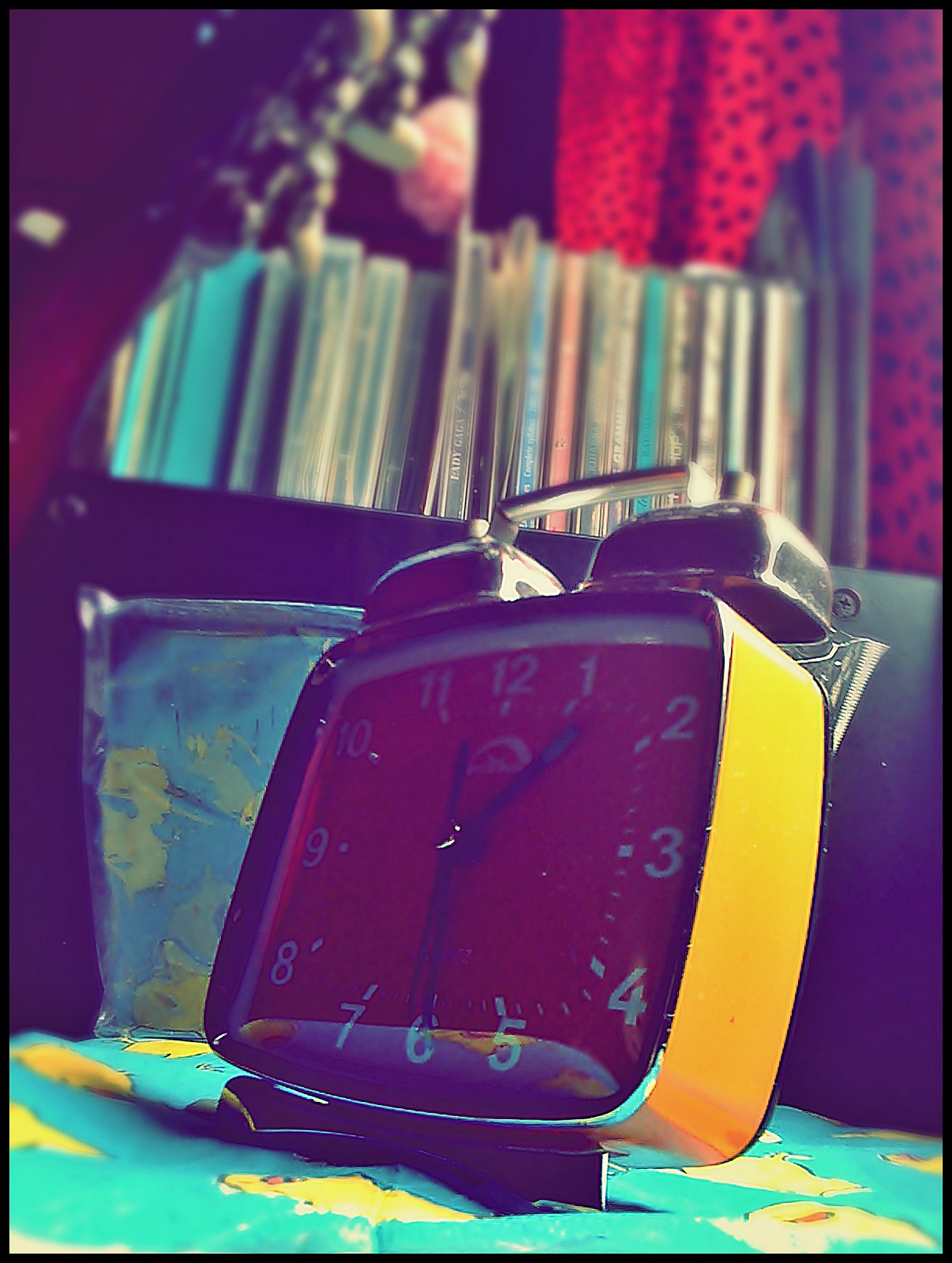The image depicts a vintage, square-shaped alarm clock with yellow sides and a red face. The clock's numbers are white, while its hands are black. The timepiece has two classic bells on top. A shadow casts over it, creating a darkened ambiance. The alarm clock rests on a turquoise surface adorned with yellow patterns, somewhat reminiscent of SpongeBob SquarePants characters. Above the clock is a bookcase filled with old books. Nearby, a clear bag reflects the turquoise and yellow design of the surface. The background features red wallpaper with purple dots and a black object situated directly behind the clock.